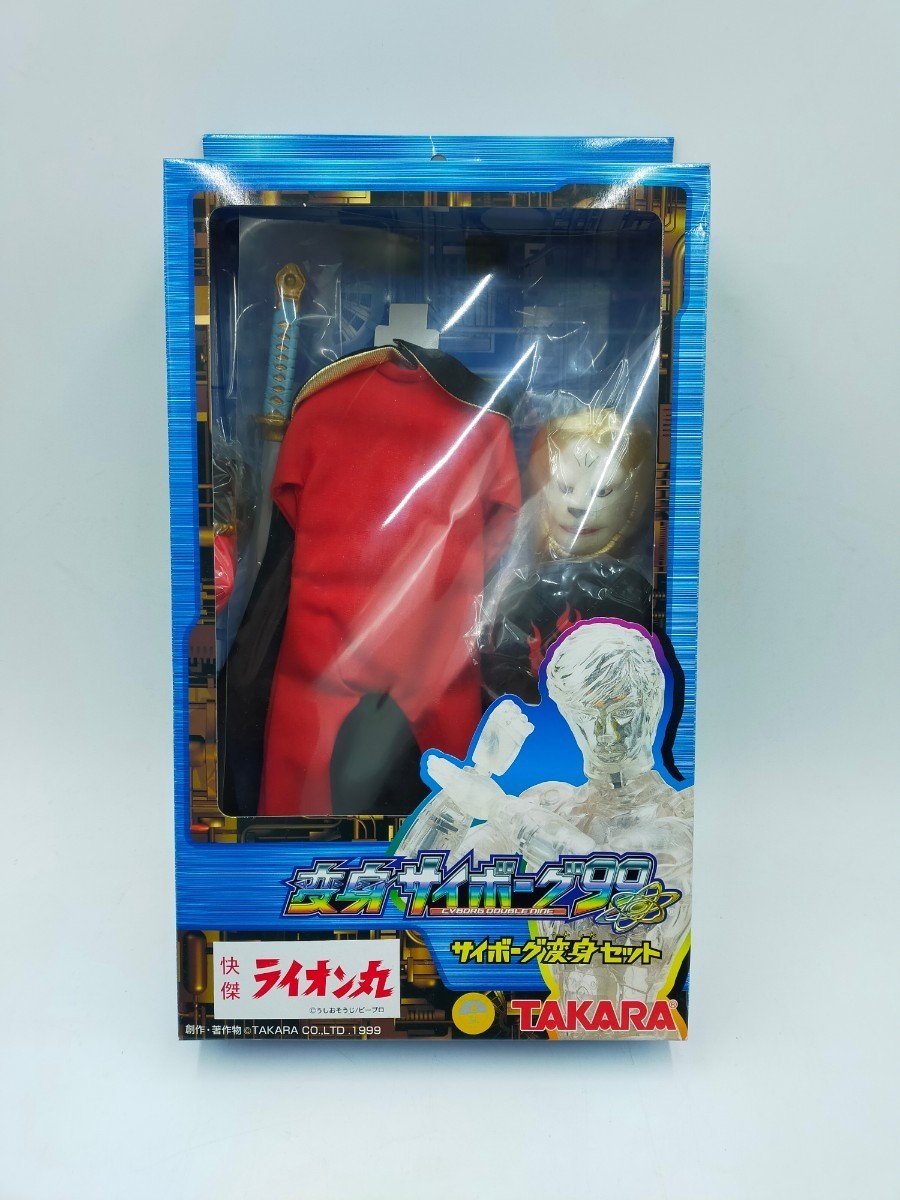The image showcases a square package with a clear plastic front on a gray background. Inside, there is a toy figure dressed in a red jumpsuit with a black cape. The toy features a lion-like face with long, blondish hair, resembling a werewolf or a dog. The toy also includes a mask with a white face and a black-tipped nose. To the right of the main figure is a section with accessories, including a sword.

The box itself is blue and prominently displays the brand name "Takara" in red text. Above this, there are Asian characters, likely denoting additional branding or product details. In the lower left corner, a small white box with red Asian text can be seen, possibly indicating a special feature or part number. There's also a crystal-like humanoid statue figure displayed on the front of the box, which appears semi-transparent and is posed holding an object, possibly a sword, with flowers in front of it.

The clear plastic packaging has some glare, making certain details hard to discern, but it's evident that this package is designed to showcase the toy and its various accessories, likely intended for display or collection.